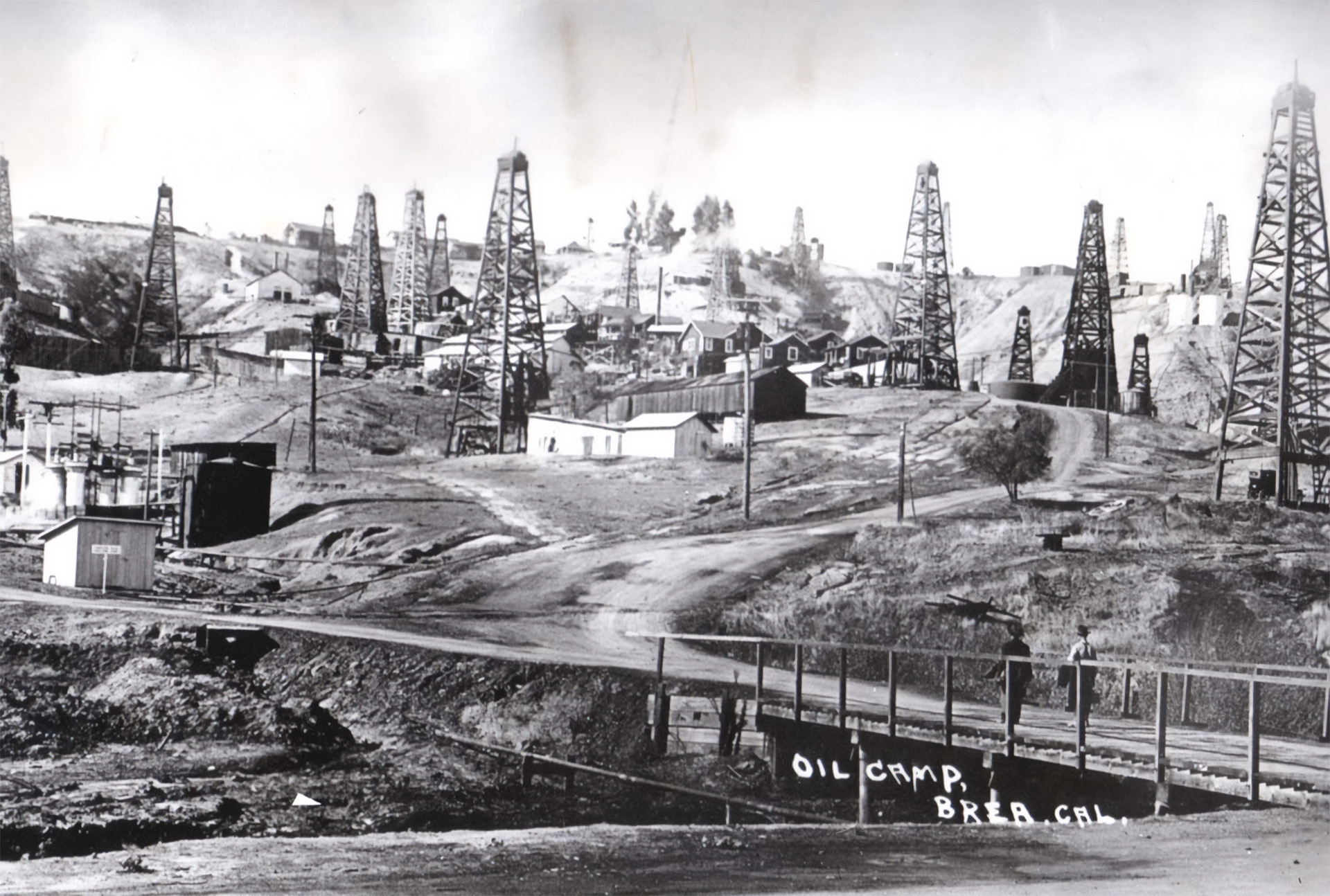This black and white image, possibly from the early 1900s, depicts a rugged oil field area known as Oyu Camp, Brea, California. The foreground features a small, wooden bridge crossed by two men in vintage attire, potentially spanning a river that is not clearly visible. Hand-written text on the lower right corner reads "Oil Camp, Brea, California." The landscape is dominated by black-gray oil towers of varying heights, from short to extremely tall structures, interspersed with shanty-like buildings and houses. The dirt roads winding through the camp illustrate the underdeveloped infrastructure of the period. The image shows a mix of elements: rough dirt paths, sprawling grassy areas, hills, and some trees. The background includes more small buildings and sheds scattered across the hills, indicating a rapidly developing area amidst the industrial boom. The sky is gray, signifying it is a daytime scene. The overall scene captures a moment in time reflective of an early 20th-century oil camp community.